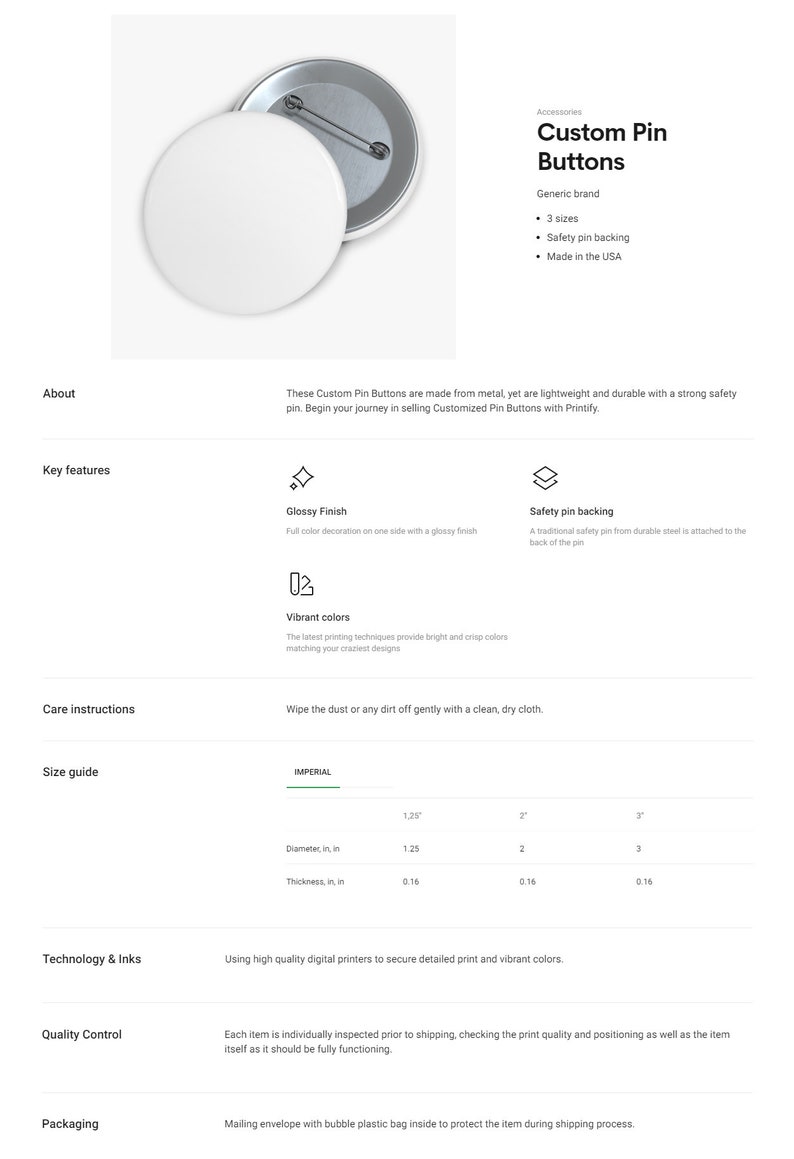Screenshot of a Website for Customizable Pin Buttons

The image depicts a screenshot of a website used for customizing pin buttons. Located at the very top left of the webpage are images of the button pins, showing both the front and back views. The front of the pins is a plain white surface, while the back reveals a silver-colored metal with an integrated safety pin mechanism.

To the right side, there is a prominent heading that reads "Custom Pin Buttons." Below this heading is an "About" section which details that these custom pin buttons are constructed from metal, making them both lightweight and durable, equipped with a strong safety pin. The section encourages users to start their journey in selling customized pin buttons with the service provider, Printfly.

Key features of the pin buttons are also listed, including:
- Glossy finish
- Safety pin backing
- Vibrant colors

Under "Care Instructions," it advises users to gently wipe off dust or dirt with a clean, dry cloth.

Although the "Size Guide" is present, the text in the chart appears too small to read clearly. Additional sections on the webpage include "Technology and Links," "Quality Control," and "Packaging," which are smaller in size and less legible in the screenshot.